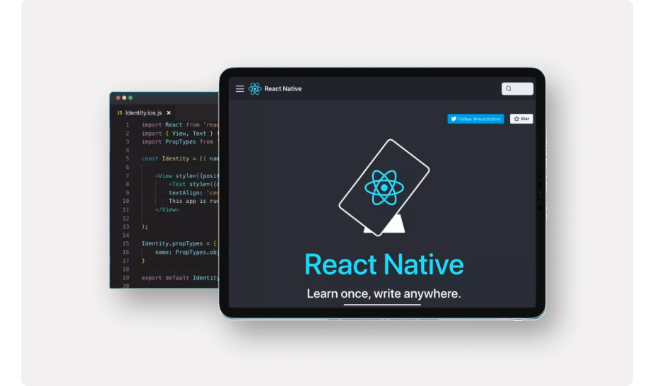The image displays a sleek and modern promotional material for React Native, viewed on a tablet. The tablet screen has a black background adorned with a central graphic resembling a scientific nucleus, featuring teal-colored spiral elements converging at the core. Prominently displayed in teal text is "React Native," followed by the tagline in white, "Learn once, write anywhere." 

In the upper right corner, there's an icon indicating the option to follow the company on Twitter. Below this, a star symbol, potentially labeled as "skill," suggests an area for skill recognition, though it's somewhat hard to decipher. Above these icons, a magnifying glass signifies a search function, and to its right, three horizontal bars represent a menu settings option.

The iconic React Native emblem, akin to a nucleus, reappears in blue near the center, with "React Native" written in white text next to it. In the backdrop, partially obscured by the tablet, is an Apple MacBook. The MacBook screen displays a script editor with code lines numbered from 1 to 20. The coding syntax includes elements in pink, blue, yellow, and orange against a black background, indicating a JavaScript file, most likely importing and utilizing React components.

Also depicted is a smartphone resting at a diagonal angle on a white base, adding to the composition's modern tech ambiance. The overall imagery suggests an environment of dynamic coding and seamless multi-device integration, reinforcing React Native's versatile development capabilities.